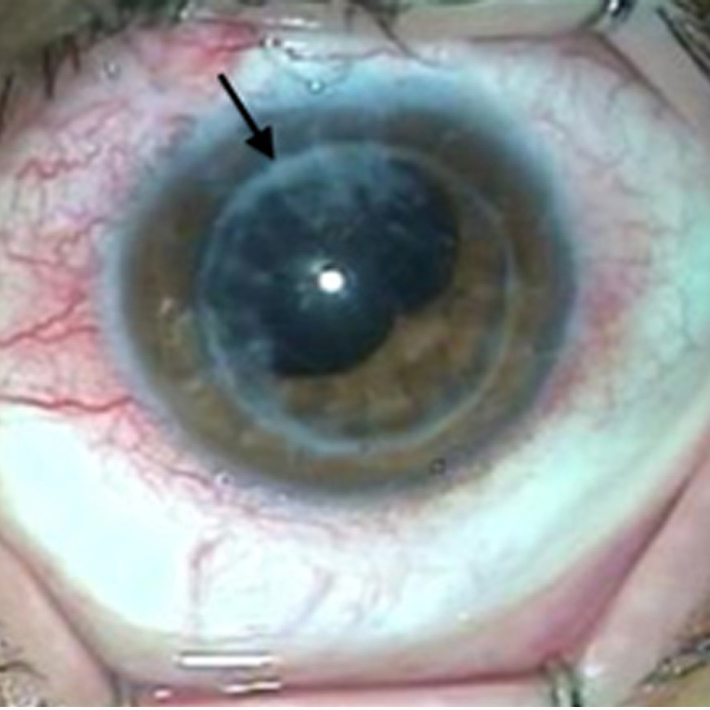This square medical photograph, approximately five inches by five inches, showcases a close-up of an eye held open by metal clamps visible in the corners, with eyelashes descending from the top. The central focus is a brown-hazel iris, which appears deformed and unhealthy. The pupil is irregular, blob-like, and positioned towards the upper left of the iris, deviating from the typical circular shape. A thin whitish-blue circle around the pupil suggests the possible presence of a contact lens; another similar outline surrounds the iris. An arrow points to the inner circle, highlighting its significance. The sclera (white part of the eye) is heavily veined with red blood vessels, particularly dense in the upper left region, giving a bloodshot appearance. The lower sclera resembles the white of an egg, while the right side is notably cloudy, indicating further possible eye health issues.